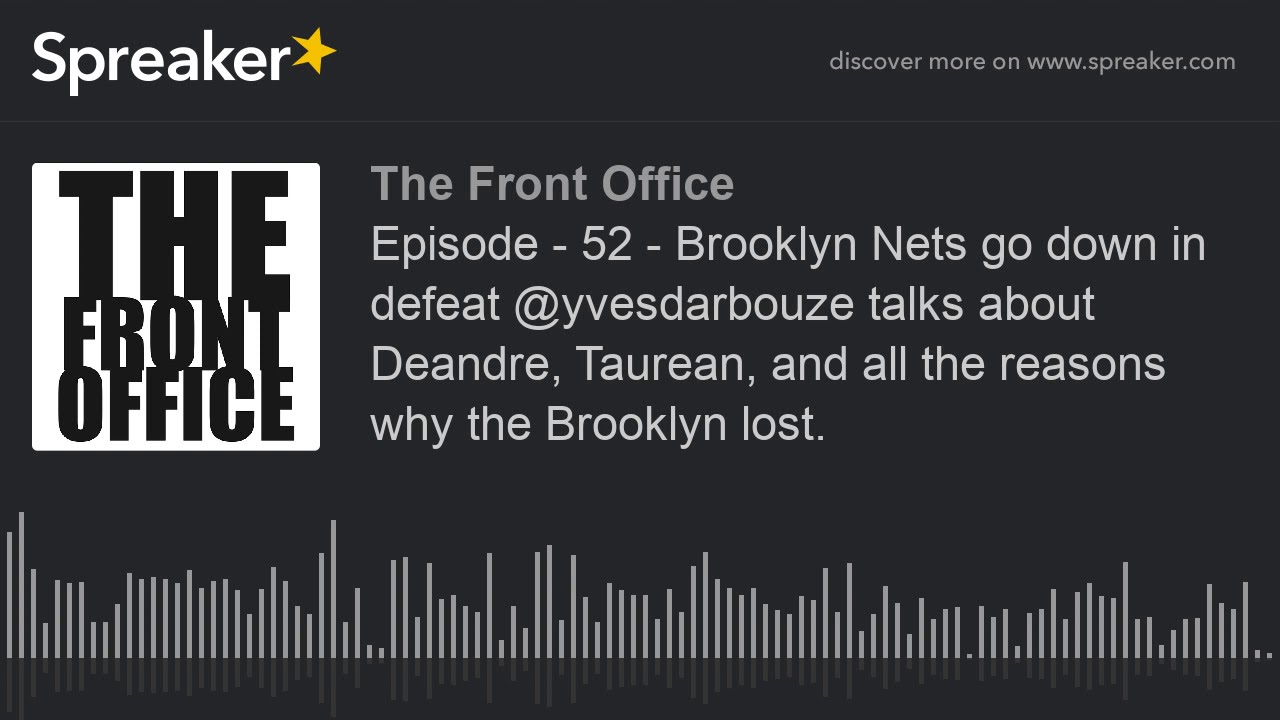This image appears to be an advertisement for a podcast episode. It features a predominantly black background. In the top left corner, the word "Spreaker" is displayed in white text, accompanied by a yellow star. On the opposite side, in smaller white font, it reads, "discover more on www.spreaker.com."

Central to the image is the title "The Front Office," repeated twice: once in black text within a white square box on the left and again in gray text beside it. Beneath the title, the caption reads, "Episode 52: Brooklyn Nets Go Down in Defeat," followed by "@YVESDARBOUZE talks about Deandre Taurine and all the reasons why Brooklyn lost." The name "Taurine" is explicitly spelled out as T-A-U-R-E-A-N.

Additionally, the bottom of the image features a series of small sound bars, akin to volume or sound wave indicators, which suggests that this is a visual representation of a podcast episode.